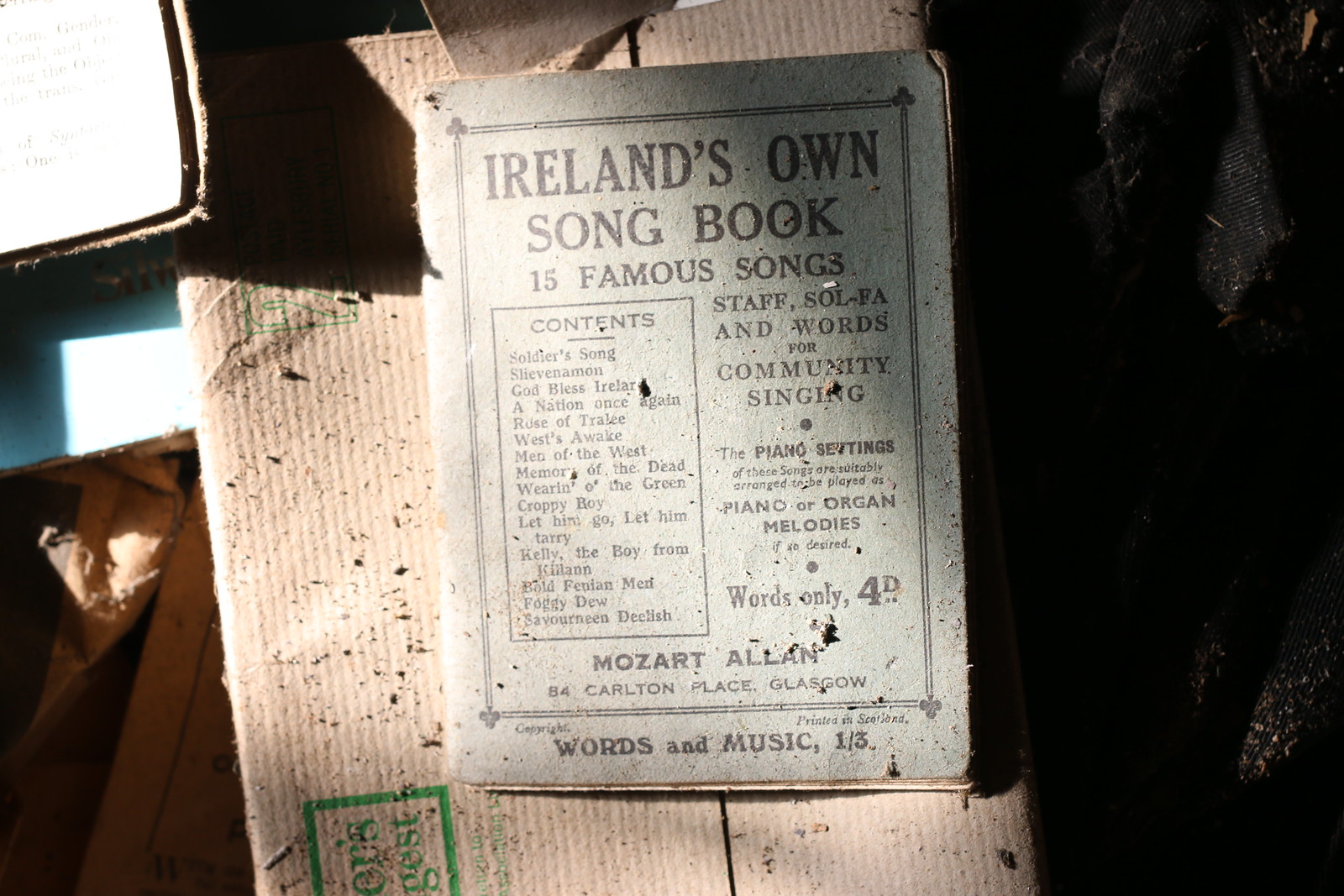This is a detailed, colored photograph of an old booklet's cover, staged indoors with light illuminating the left side while the right remains in shadow. The bluish-green paper cover, showing signs of significant wear and age such as fraying and debris, prominently displays the title "Ireland's Own Songbook, 15 Famous Songs". The text, enclosed within a blue border, includes details like "Contents" on the left, "Staff and Words for Community Singing" on the right, and a list of song titles such as "Soldier's Song," "God Bless Ireland," and "A Nation Once Again." The bottom section features "Mozart Allen, 84 Carleton Place, Glasgow" and "Words and Music, 1/3." The book, likely from the late 1800s or early 1900s, sits on a cardboard box, adding an antique atmosphere to the composition.